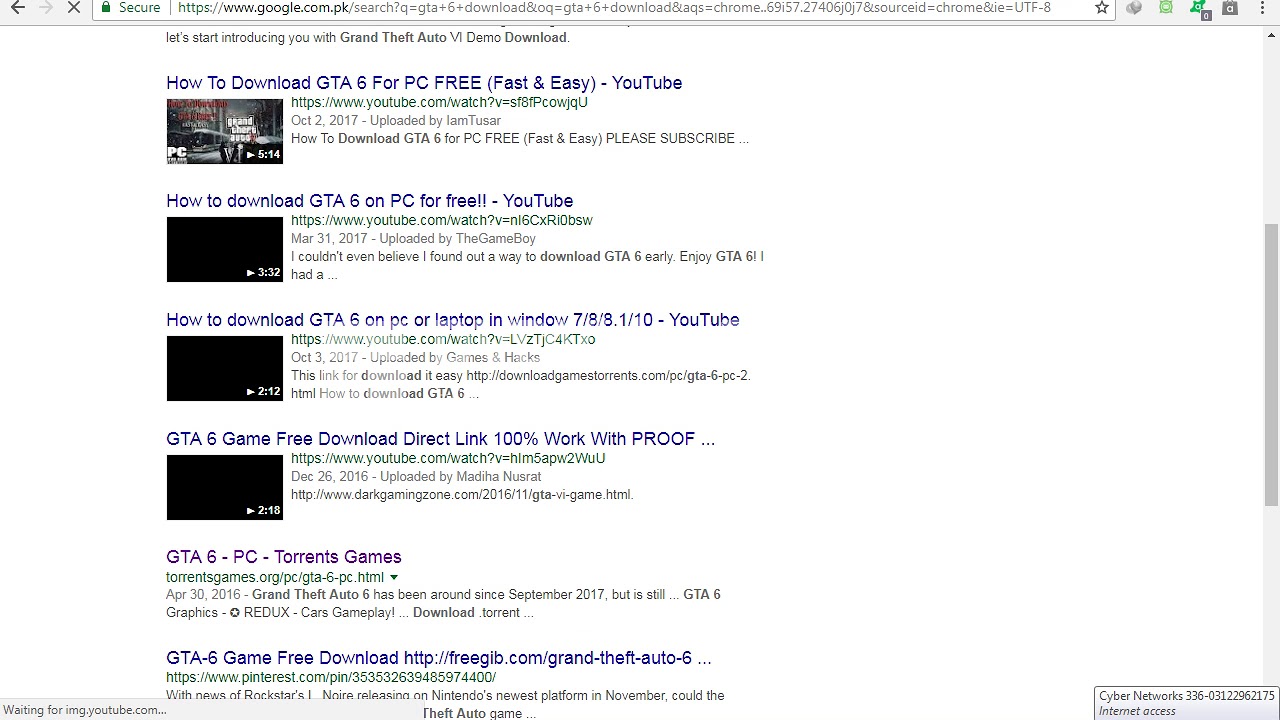The image is a horizontal screenshot of a web browser window with a white background. Along the right-hand side, there is a gray vertical scroll bar. A light gray banner is located at the top, featuring a left-pointing arrow and an 'X' button. The lower left-hand corner of the browser indicates an ongoing web search with the message, "waiting for img.youtube.com." An address has been entered into the search bar at the top. 

In the upper right-hand corner, several small icons are visible. Below the search bar, search results are displayed in bold blue font, functioning as clickable links that redirect to different websites or search suggestions. There are four horizontal video boxes—one at the top with a thumbnail image, and three below that display a black screen.

The search results shown include:
1. "How to download GTA 6 for PC free, fast and easy - YouTube"
2. "How to download GTA 6 on PC for free L - YouTube"
3. "How to download GTA 6 on PC or laptop in Windows 7, 8, 8.1, 1, 10 - YouTube"
4. "GTA 6 game free download direct link 100% work with proof"
5. "GTA 6 PC torrents games"
6. "GTA 6 game free download"

The link "GTA 6 PC torrents games" appears in purple, suggesting that the user has previously clicked on this link while searching for videos related to downloading GTA 6 on YouTube.